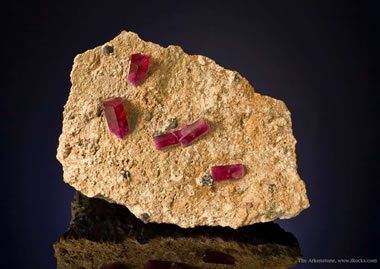The image showcases a prominently positioned tan geode rock, meticulously cut in half to expose its inner beauty. Occupying approximately three-quarters of the frame, this misshapen rock, with its natural curves and jagged edges, reveals four to five bright red gemstones set in a zigzag pattern from left to right. The gemstones, resembling dark red rubies, add a striking contrast to the rock’s tan coloration. Scattered black dots are visible within the rock, which appears solid and non-porous. The geode rests on a shiny black surface that mirrors its reflection, accentuating its form. The background is a nearly black expanse, subtly tinged with a very dark blue hue towards the center. A small white text label is discreetly placed in the bottom right corner of the image, providing a minimalistic yet informative touch.